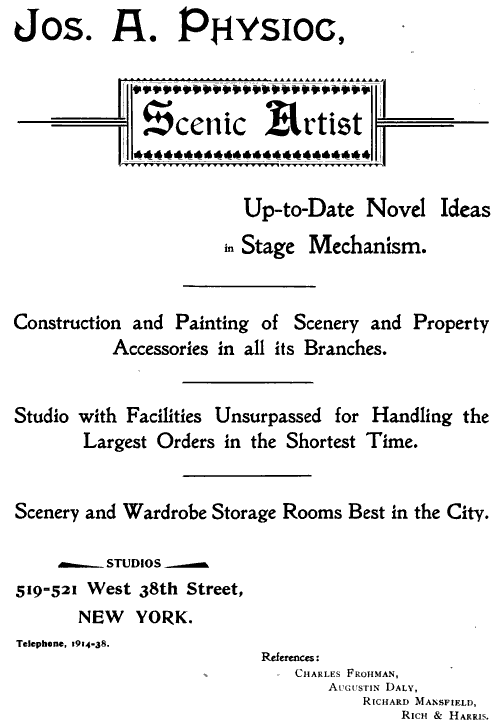The image showcases a meticulously arranged, black-and-white printed document, predominantly focusing on text. At the top, the text "J.O.S. A. PSYOC" is prominently displayed, identifying the individual as a "Scenic Artist." The document, resembling a business advertisement, highlights Jos A. Psyoc's expertise in "Up-to-Date Novel Ideas and Stage Mechanism," and offers services in "Construction and Painting of Scenery and Property Accessories in All its Branches." It emphasizes the studio's superior facilities which are "unsurpassed for handling the largest orders in the shortest time," along with having the "best in the city" for scenery and wardrobe storage rooms. Located at "Studios 519, 521, West 38th Street, New York," the document provides contact information with a telephone number "1914-38." At the bottom, it lists references: Charles Froman, Augustus Daly, Richard Mansfield, and Rich and Harris, suggesting notable endorsements. The text is well-positioned and easy to read, with distinct sections separated by lines, giving it a clean and professional appearance.